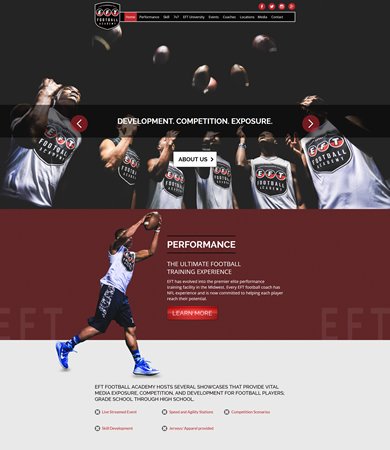This image showcases an advertisement for EFT Football Academy, emphasizing its comprehensive football training program. The ad prominently features the phrases: "Development," "Competition," "Exposure," "About Us," "Performance," and "The Ultimate Football Training Experience," suggesting a well-rounded approach to enhancing football skills.

The focal point includes a "Learn More" button positioned below a dialogue box labeled "About Us," encouraging viewers to explore further details about the academy. At the bottom of the ad, additional text highlights that EFT Football Academy hosts numerous showcases designed to provide vital media exposure, competition, and developmental opportunities for student-athletes ranging from grade school through high school. This suggests that the academy not only focuses on improving players' football skills but also aims to increase their visibility in the media, potentially aiding those seeking a professional career in football.

Overall, the design and content of this advertisement are crafted to attract aspiring football players and their families, portraying EFT Football Academy as an elite training destination that goes beyond standard personal training to offer a pathway to greater recognition and success in the sport.